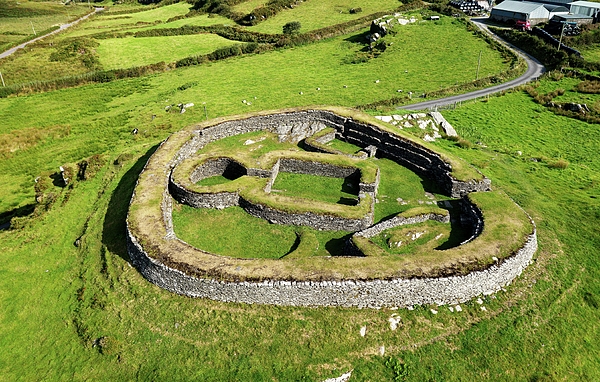The photograph depicts a large, hilly expanse of light green grassland, possibly situated in the rural areas of Scotland or Ireland. Dominating the center is an ancient, somewhat circular structure made of grayish stone, resembling ruins from the Iron Age or Neolithic period. This circular design features two concentric stone walls with patches of dirt and sporadic grass growing in between, creating what could be considered a raised flower bed. Within this main circle lies an internal, keyhole-shaped configuration crafted similarly from stone, with two walls enclosing it. The keyhole shape leads to a narrow opening that transitions into a larger, square enclosure, both also bordered by stone. Surrounding the site are green fields and some bushes, emphasizing its rural and historical setting. In the background, a winding road connects the structure to a cluster of barns situated in the top right-hand corner of the image. This site, with its enigmatic shapes and stone constructs, is a striking remnant of ancient architecture, evocative of historical sites found in the British Isles.